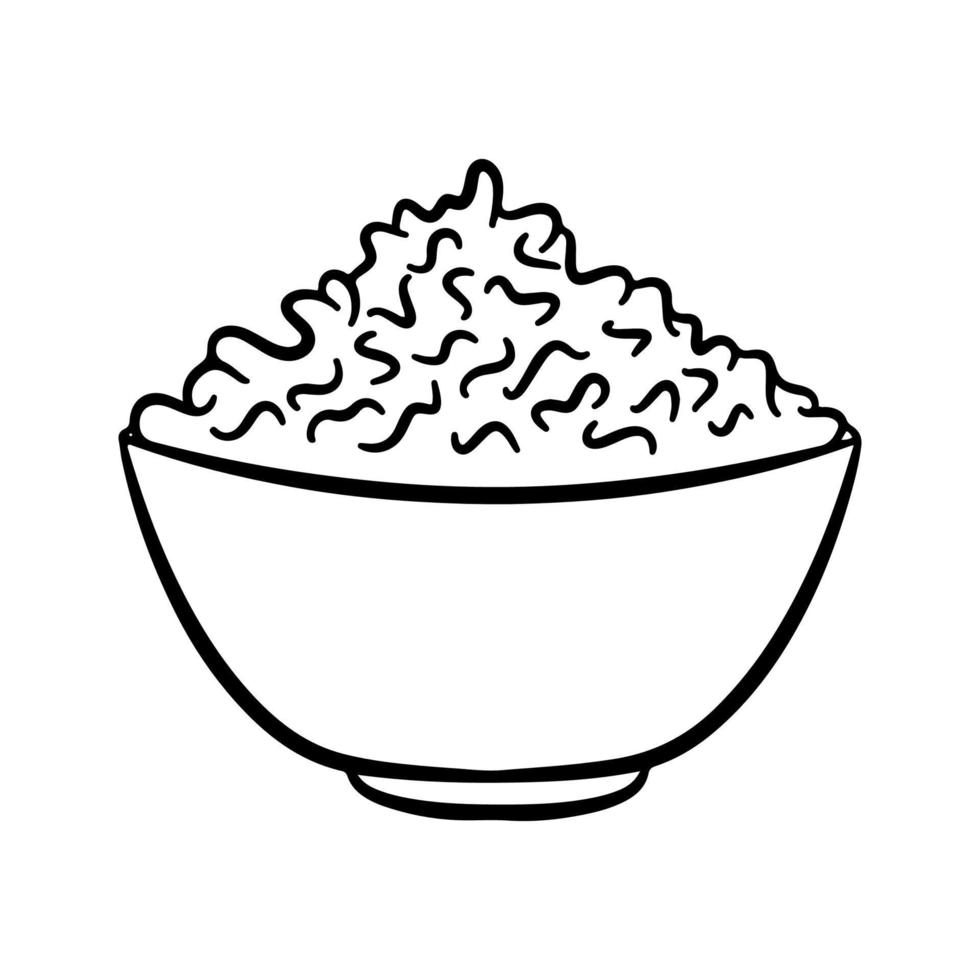This is a detailed black-and-white illustrated image featuring a simple and stylized bowl of food, possibly noodles, rice, pasta, or even cereal. The bowl is plain with a small base at the bottom and is centered in an entirely white background. The contents of the bowl are represented by various squiggles and lines, forming a triangular mound of food. The sketch uses only outward lines to depict the food, making it somewhat ambiguous yet suggestive. The overall minimalistic design of the image gives it an iconic feel, devoid of any text or additional elements.